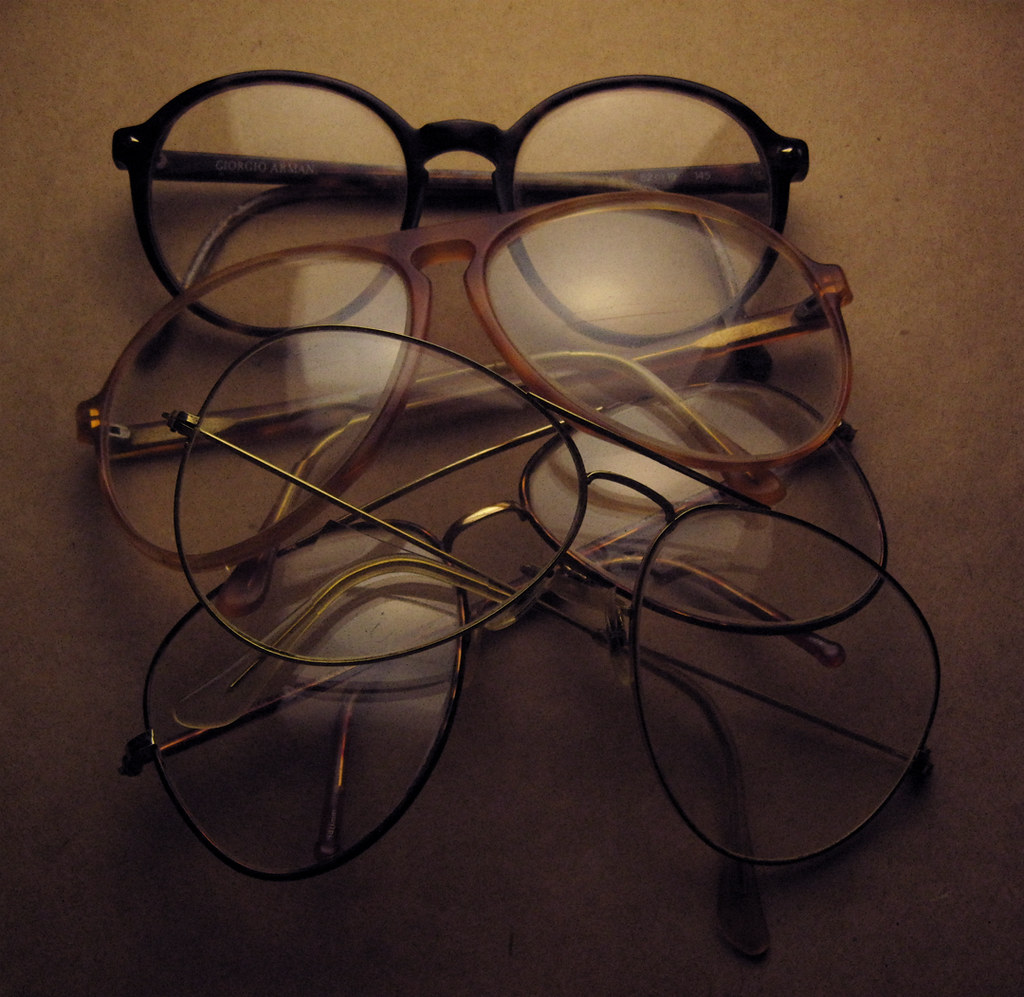The photograph showcases a stack of four pairs of reading glasses arranged in a layered, somewhat haphazard manner on what appears to be a brownish-tan surface, possibly mimicking a cardboard table. The topmost pair features circular black plastic frames with the words "Giorgio Armani" faintly visible in white lettering on the temple arm. Nestled directly below are glasses with bold red plastic frames. The third pair stands out with a tortoiseshell or cheetah-like brown pattern, while at the base are two pairs of classic wire-framed glasses, their delicate designs suggesting vintage sophistication. The glasses' transparent lenses and the descending shadow gradient from light at the top to darker at the bottom give the photo an artistic flair.